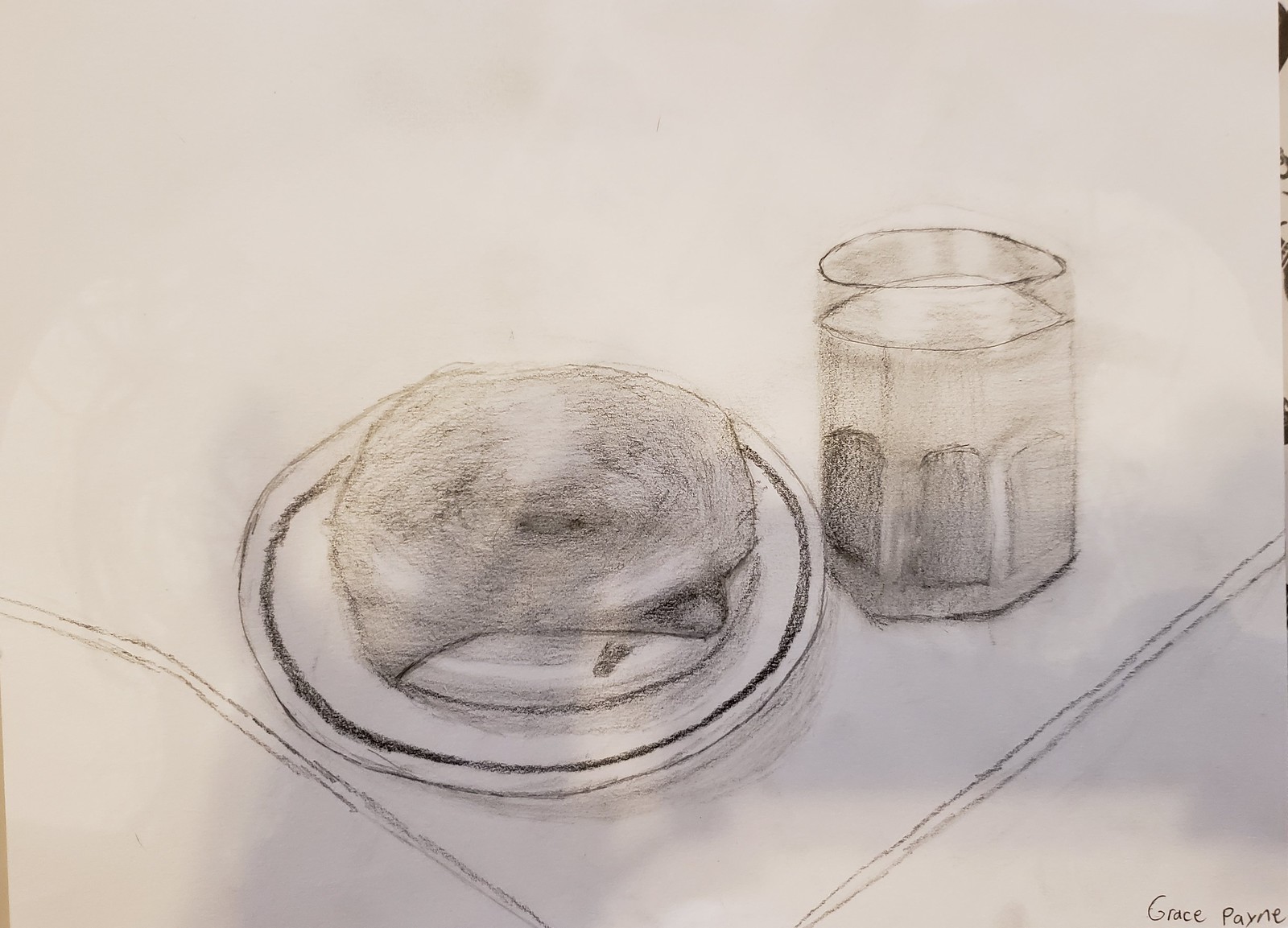This highly detailed pencil drawing by artist Grace Payne depicts a meticulously rendered sandwich placed on a round plate with a distinct, dark stripe encircling its border. The plate is accompanied by a clear glass featuring subtle textures along its sides, suggestively filled with water due to the transparency of the liquid inside. Situated beyond the plate and glass, the composition includes a delicately drawn edge that subtly implies the presence of either a placemat or a piece of paper beneath the arranged items. The drawing is executed on lightweight, unbleached, and naturally tinted paper, adding to its organic aesthetic. The artwork is personally signed by the artist, Grace Payne, lending an authentic touch to this exquisite piece.